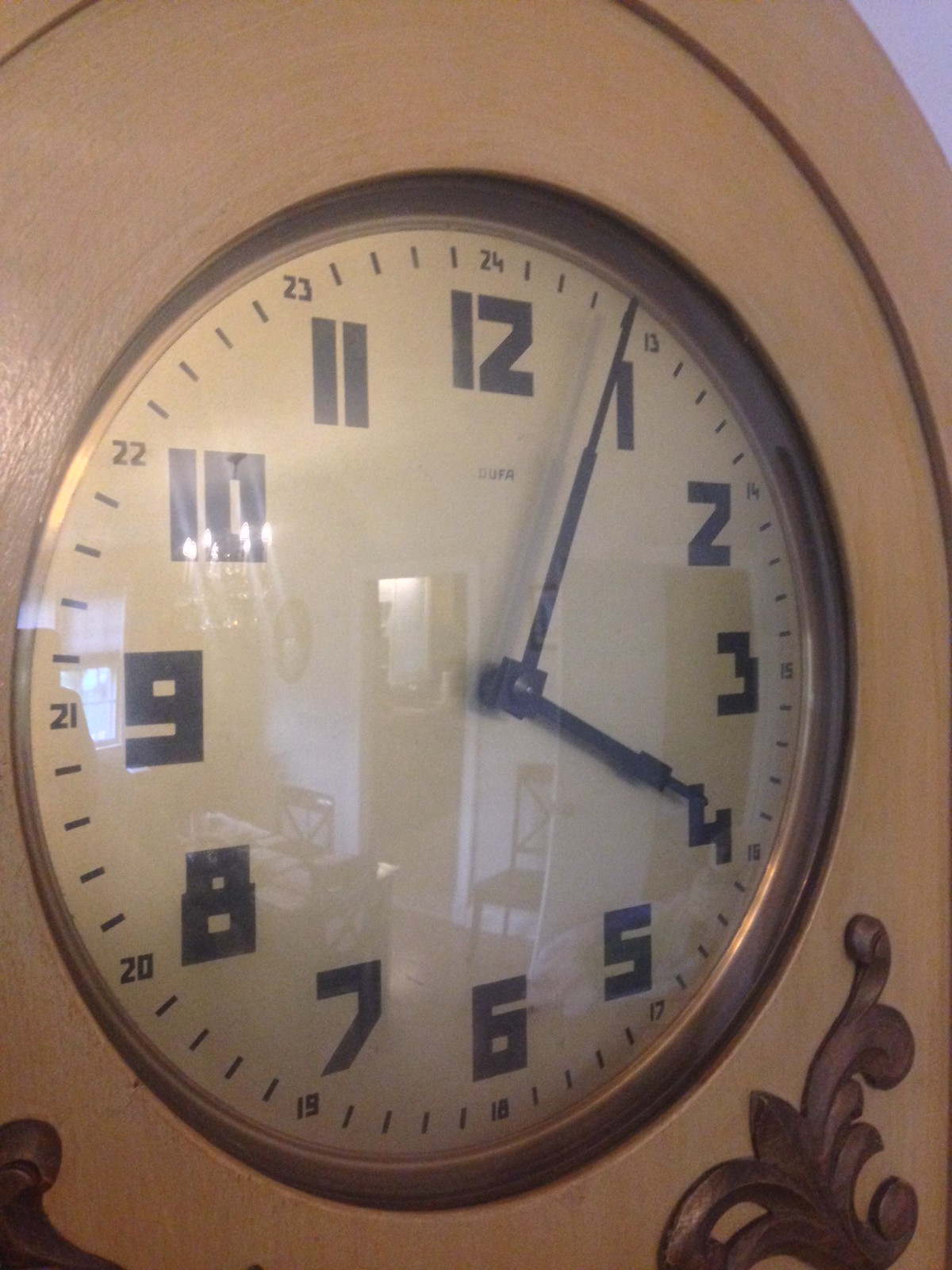This photograph captures a close-up view of a wall-mounted clock, showcasing its ornate and detailed design. The clock is encased in a thick frame that appears to be made of wood, possibly with a copper or golden hue. The frame features two substantial rings separated by a distinct line, with the bottom adorned by intricate dark-stained wood or bronze-like ornamental designs resembling fleur-de-lis patterns. The clock face itself is white and covered by a glass or plastic bubble, which reflects the interior of the house.

The clock numbers are thick and black, set in a retro sci-fi font. Each number from 1 to 12 is accompanied by smaller military time indicators, making it easy to read both standard and military time. Below the black number 12, there is a small text that seems to spell out "DUFA." The black clock hands point to slightly past 4:00, suggesting the time is around 4:05 PM.

In the reflective surface of the clock cover, various elements of the house interior are visible. This includes a dining room with hardback chairs, a wooden table, light blue walls, and a chandelier. The reflection also shows a doorway with white trim leading into another room and a window, hinting at a cloudy day outside.